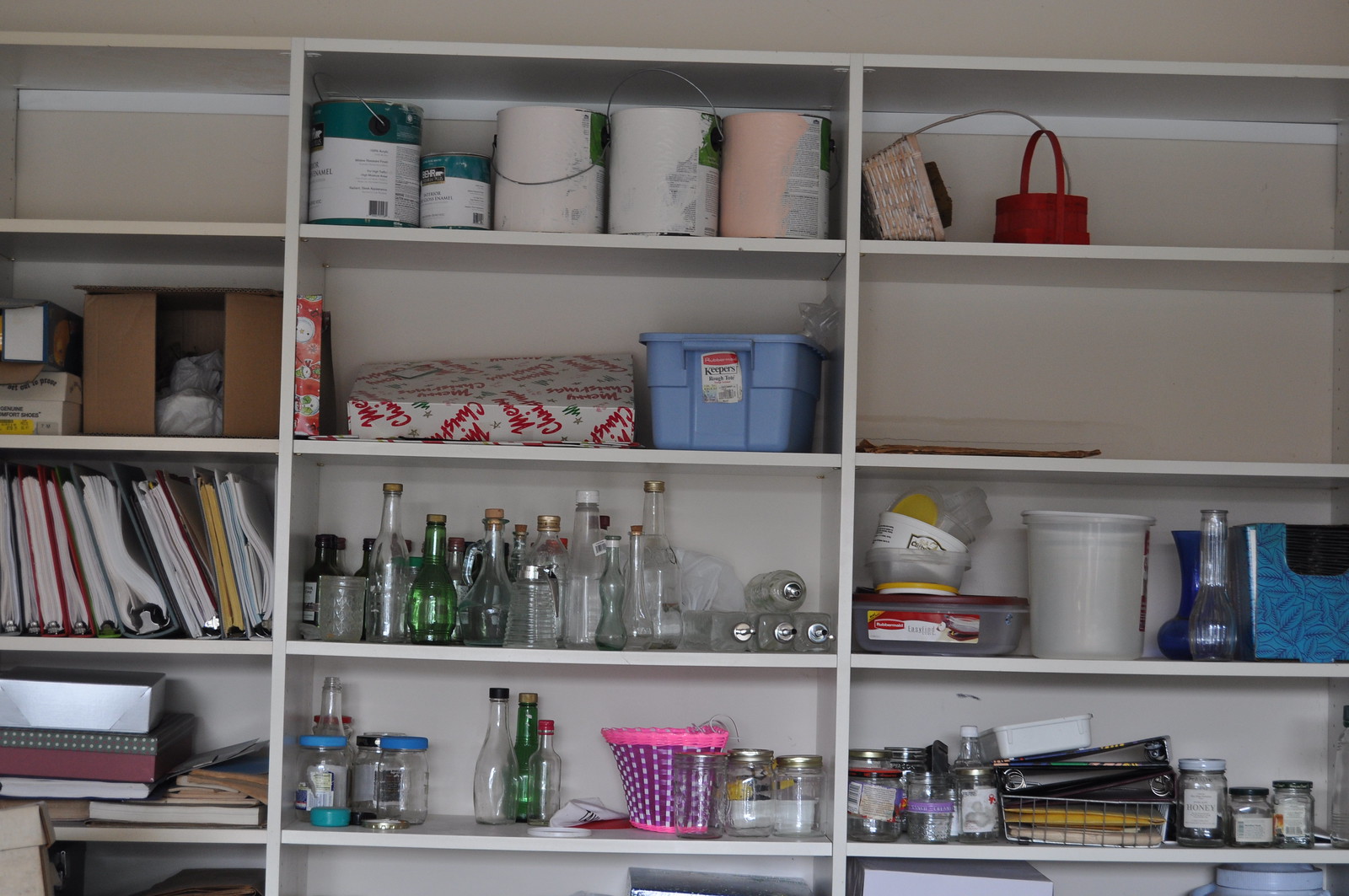This image depicts a multi-compartment shelf, resembling a large closet organizer commonly found in a typical home. The shelf has approximately 12 visible compartments, primarily rectangular, with a variety of items stored within them. Though the bottom section of the image is partially obscured, the contents of the upper compartments are clearly visible.

Starting from the top left, the first compartment is empty. Below it, the second compartment houses a brown cardboard box along with a few miscellaneous items. The third compartment contains several binders and books. Directly underneath, the fourth compartment holds a few boxes, possibly shoe boxes, with an additional book.

Moving to the middle section, the first compartment features multiple cans, possibly tins or cylindrical containers, though their contents are unclear. Below, there are two boxes wrapped in Christmas paper, suggesting they might be presents, along with a blue Sterilite storage tote. Underneath that, various glass bottles, all empty and corked, are neatly arranged. Further down, the next compartment also has more glass bottles and a pink and purple basket.

Onto the far-right section, the first compartment shows a handbag accompanied by another basket. Directly below this, there is a piece of paper, potentially an envelope, though it is not distinctly visible. The adjacent shelf houses a wastebasket, a couple of additional items, and a food container paired with a random bottle. Finally, the last completely visible shelf in the middle section contains several binders and various glass jars.